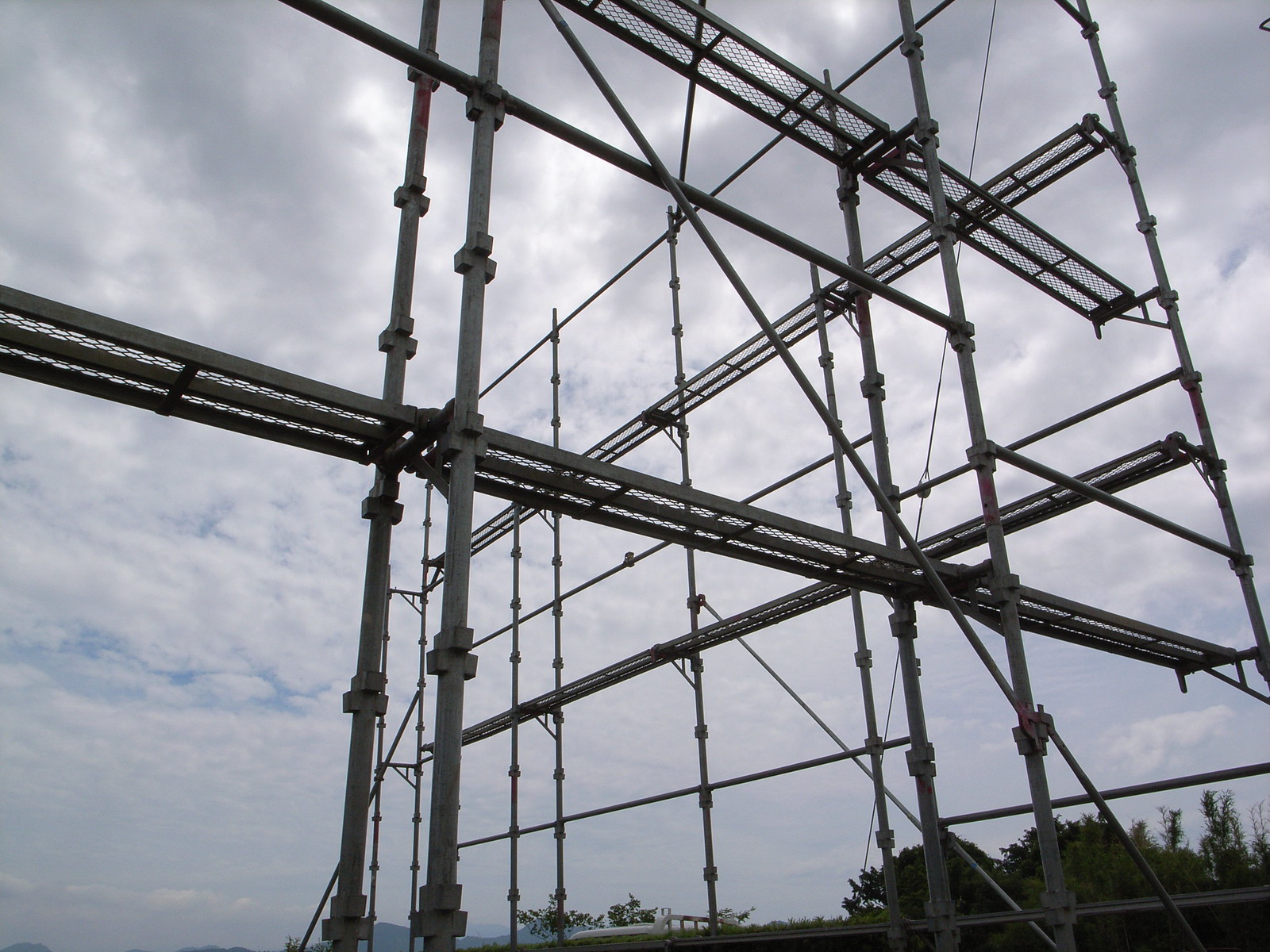The image depicts an outdoor scene dominated by a large, black, steel scaffolding structure with multiple levels intended for construction work. This intricate network of metal beams and walkways spans across the image, offering various paths for workers to navigate, highlighted by a central path and higher levels. The overcast sky, filled predominantly with white clouds and occasional glimpses of blue, sets a dim tone for the scene. In the background, a white-topped building and some trees, which rise to the lower part of the scaffolding, add depth to the composition. Light fog can also be discerned in the air, contributing to the moody atmosphere. Despite its imposing height and industrial appearance, the structure is devoid of any visible workers, underscoring the formidable and somewhat precarious nature of this construction site.